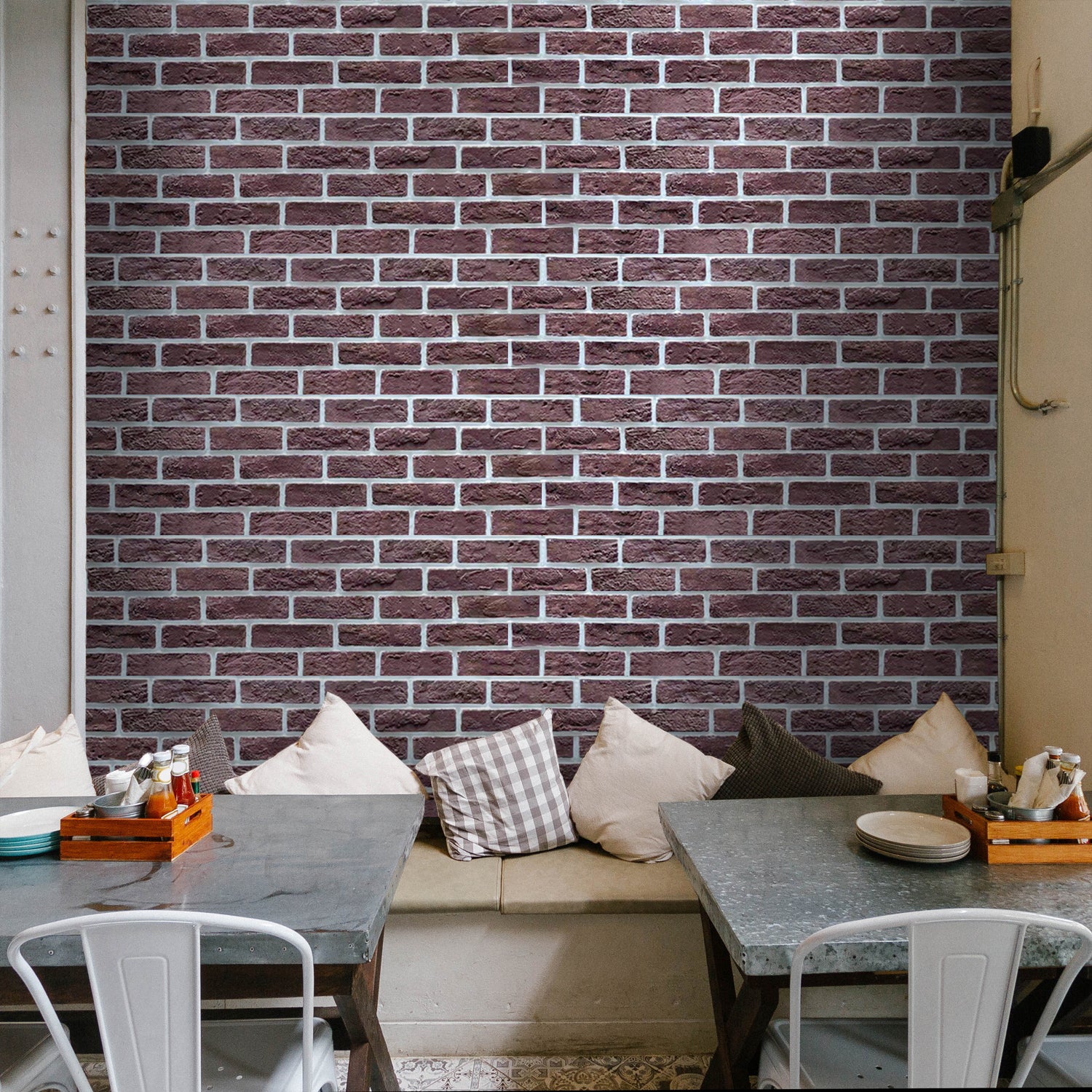The image depicts a cozy nook inside a cafe or shop. Dominating the background is a dark brown brick wall with white grout, each row of bricks meticulously counted, topped with a row of 11 bricks. To the left, a white-painted steel beam with eight visible rivets frames part of the scene, while to the right, metal casing encloses wires leading up through the walls. Below the brick wall sits a padded bench with a beige seat and decorative throw pillows—four white, two dark gray, and one gray and white checkered. The lower part of the picture also reveals a decorative white tiled floor. 

In front of the bench are two square tables, each with brown legs and gray marble stone tops. These tables are adorned with brown trays holding ketchup and mustard bottles, silverware, and small stacks of white plates. Complementing this setup are modern white metal chairs, suitable for a casual yet stylish indoor setting. Overall, the scene balances industrial elements with cozy touches, making it an inviting spot within the larger cafe.